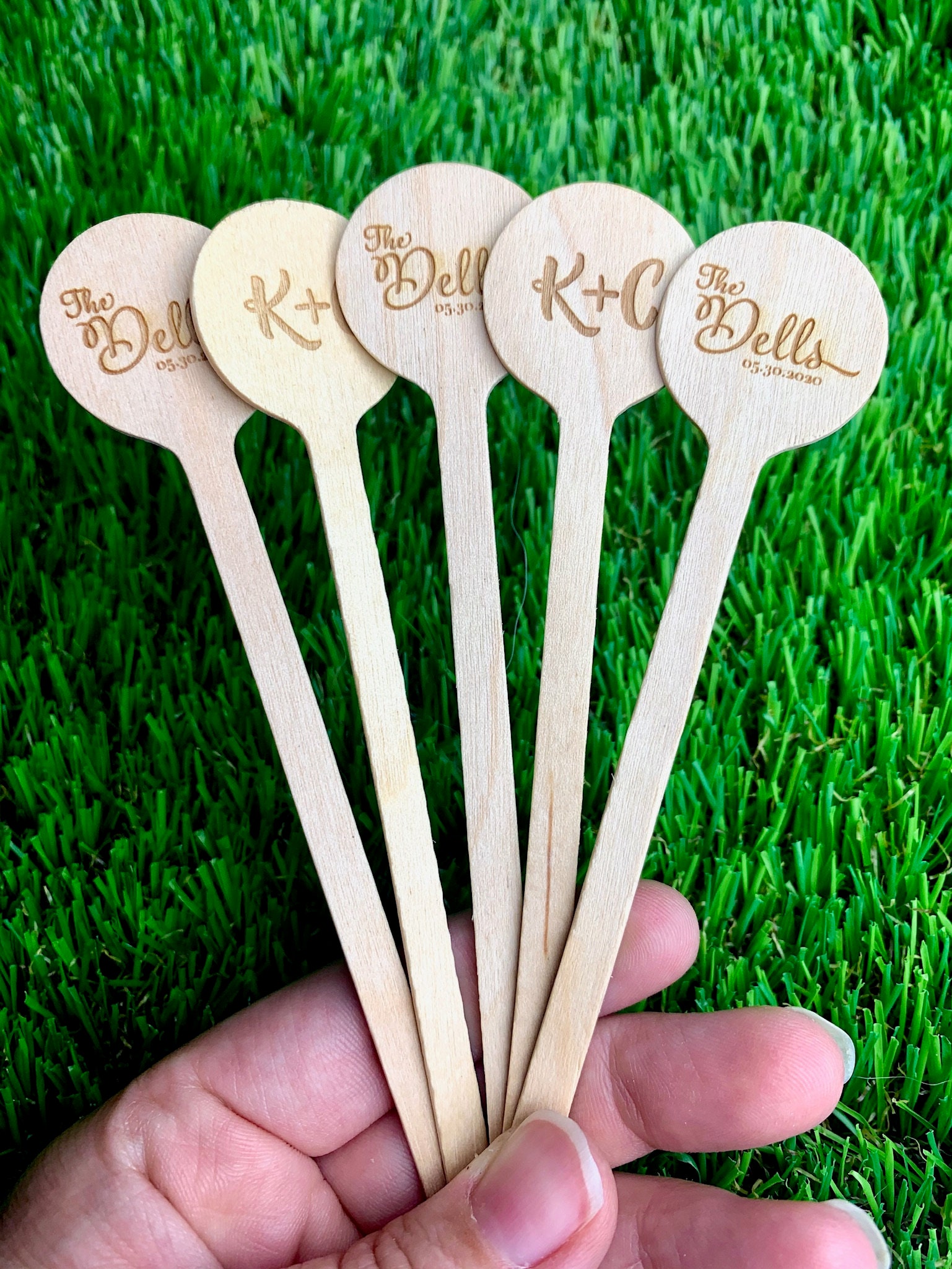In a verdant, grassy setting, a person's left hand—belonging to someone of Caucasian descent, possibly a man or a woman—delicately holds five slender wooden sticks that resemble coffee stirrers. Despite concerns about the wood's potential reaction to coffee, they seem better suited as charming placeholders for a wedding. Each stick bears inscriptions: "The Dells," possibly alluding to Wisconsin Dells as the wedding location, "K & C," which could be initials of the couple, and the date "May 30th, 2020." These personalized touches suggest the sticks are likely used as wedding favors or decorative items intended to add a personal, rustic touch to the event.